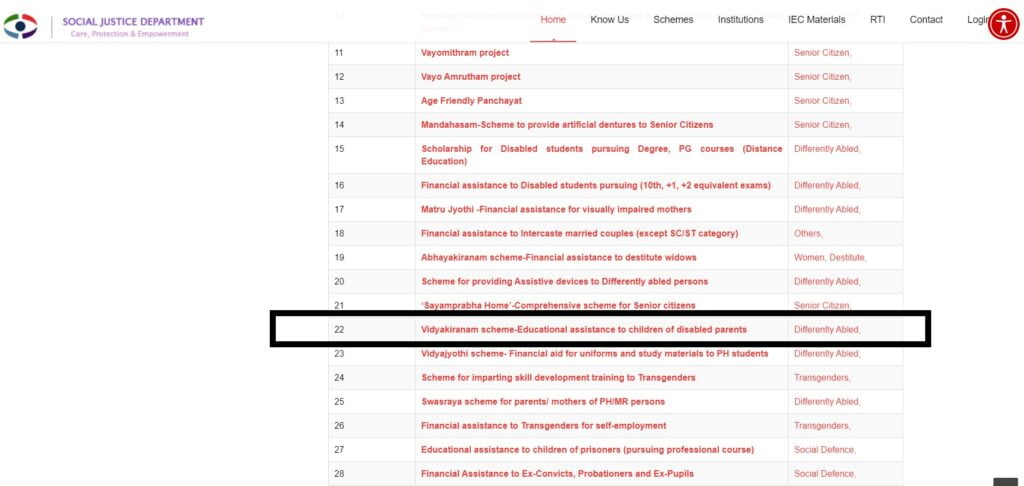The image features a white screen displaying a spreadsheet that lists items numbered 11 through 28. Notably, item number 22 is highlighted with a bold black rectangle. The central column, written in red text, reads: "Vidya Akiranam Scheme Educational Assistance to Children of Disabled Parents Differently Abled." In the upper left-hand corner, there is a multicolored logo resembling an eye, accompanied by purple text that reads: "Social Justice Department Care Protection and Empowerment." Adjacent to this title is a menu, and in the upper right-hand corner, a red circle with an icon of a person in the center can be seen. The middle column lists the names of different projects, while the first column contains the item numbers, and the last column includes additional specifications about each project.